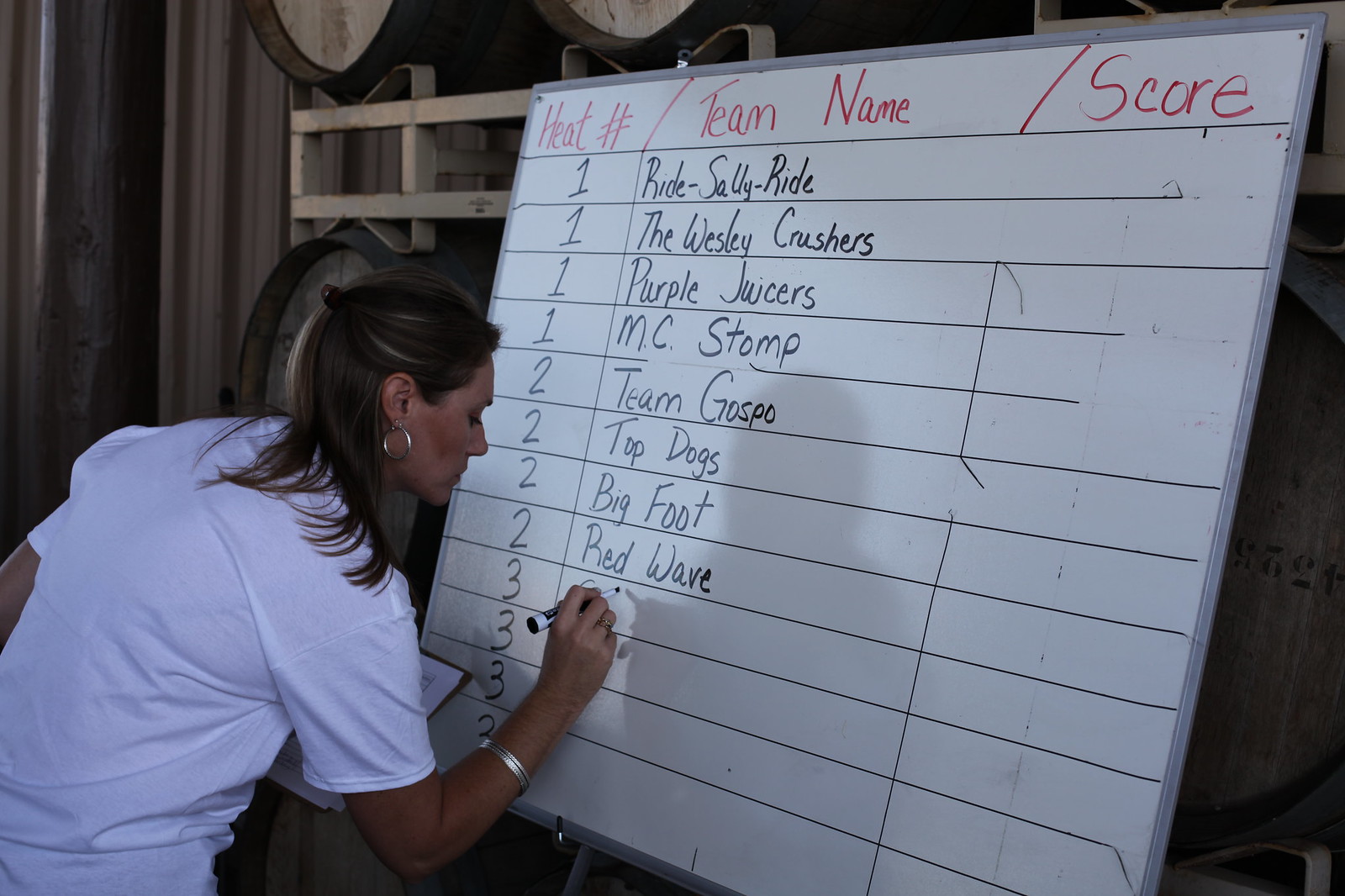In this detailed photograph, we observe a woman meticulously constructing a scoreboard on a whiteboard set up on an easel. The whiteboard is organized into three columns—Heat Number, Team Name, and Score—to keep track of an event's progress. The woman appears to be in her mid-30s to early 40s, sporting a half-ponytail with highlights in her hair, large silver hoop earrings, and a white t-shirt. She's also adorned with a platinum gold bracelet on her right arm, which she is using to write. In her left hand, she holds a small clipboard.

The Heat Number column is broken down into four sequential sets, and the Team Name column is being populated with names of the competing teams. So far, the list includes: Ride Sally Ride, The Wesley Crushers, Purple Juicers, MC Stomp, Team Gospo, Top Dogs, Bigfoot, and Red Wave. The Score column remains empty at this stage. The woman is actively writing the first line of the third heat at the moment the photograph was taken.

In the background, wine or distillery racks holding large barrels suggest that the event might be taking place at a winery or a similar venue. The woman is almost fully turned away from the camera, revealing her elegant, flowing handwriting on the board.